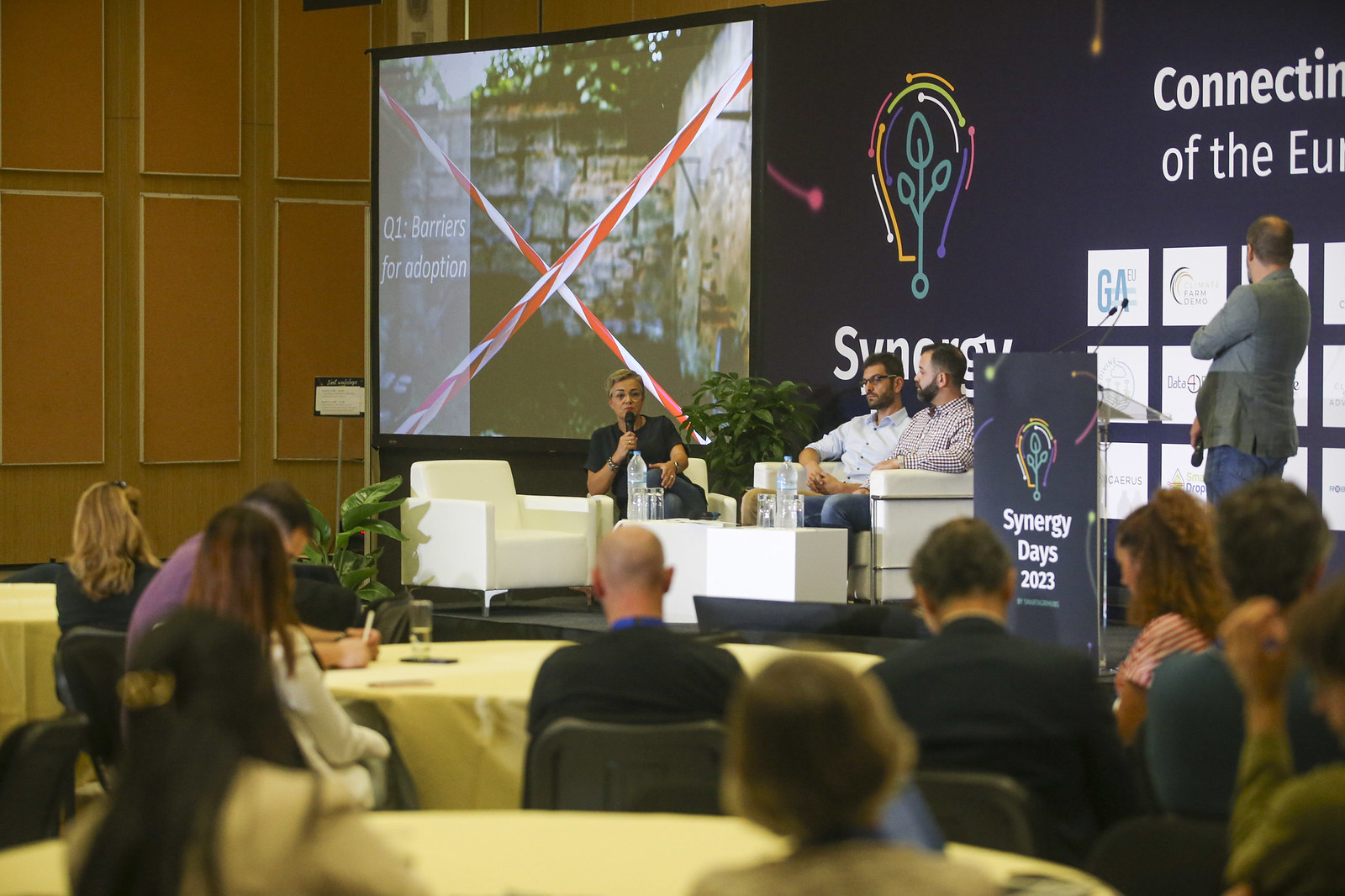The image showcases a conference-style panel discussion taking place on a stage adorned with the Synergy Days 2023 branding. Centered on the stage are three white chairs, including a love seat occupied by two men, and a single chair to the left with a woman in a black shirt with short hair, who appears to be the moderator holding a microphone. Behind them, an individual with a gray jacket stands, also holding a microphone. The backdrop features a large screen displaying "Q1 Barriers for Adoption" in italicized white text, partially obscured by crisscrossed white and red streamers or strings resembling an X formation. The screen also prominently features the Synergy logo—a white light bulb illustration with teal leaves sprouting inside. The audience, seated at round banquet tables, faces the stage, indicating an interactive symposium or keynote discussion setting.